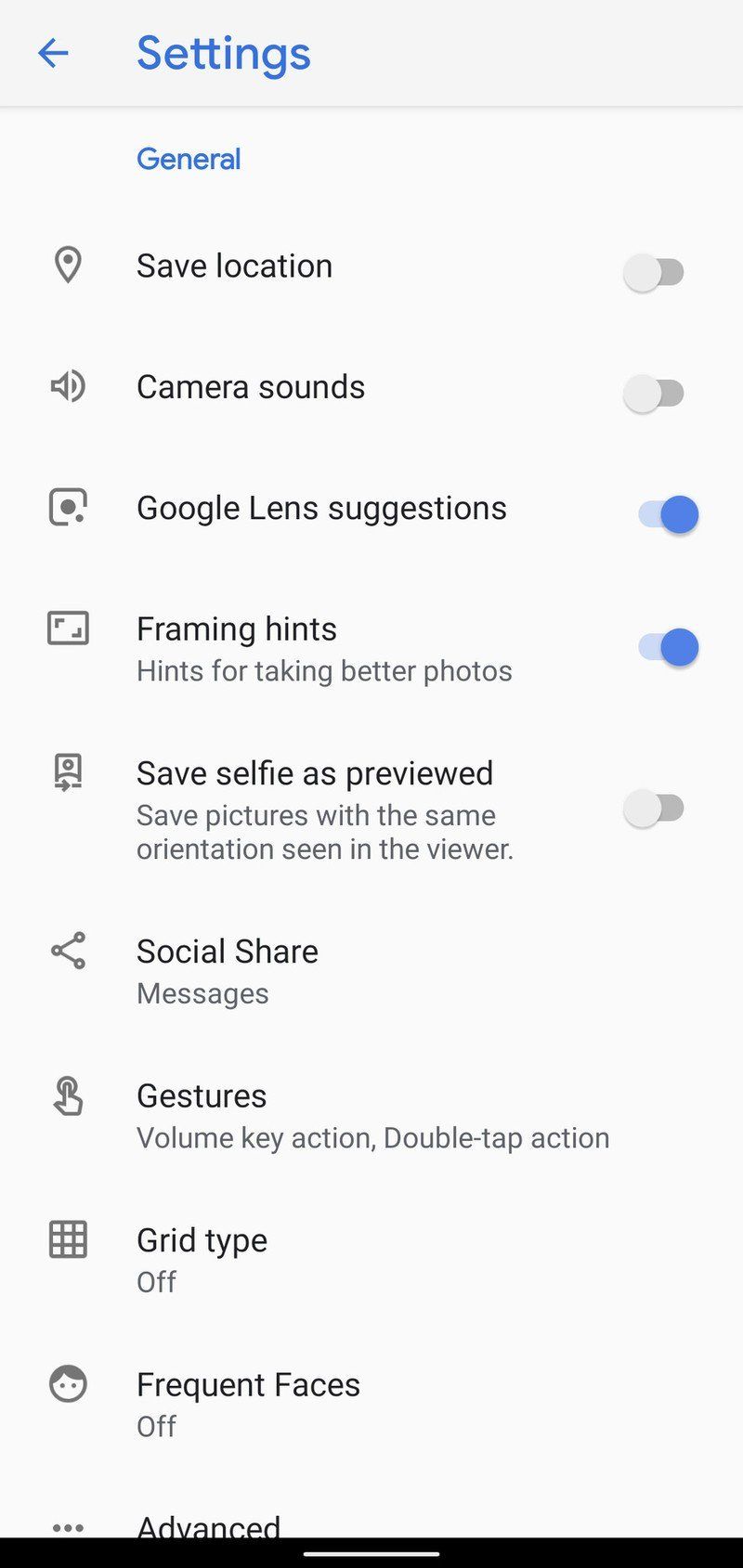At the top of the image, there's a gray header box featuring a blue, left-pointing arrow next to the word "Settings" in large blue letters. Directly below this, a darker gray line separates the header from the rest of the content. The first section underneath includes "General" highlighted in blue, paired with an icon indicating a map location to its right. Adjacent to this, the words "Save Location" are displayed beside a button with an inactive slider.

Following this is a section including a camera or sound icon paired with the label "Camera Sounds" and another inactive slider button next to it. The next part displays a box with a pair of dots labeled "Google Lens Suggestions," and its corresponding slider is blue and active, indicating that it's shifted to the right.

Further down, there's a frame logo icon next to the text "Framing Hints," and below this, a description that says "Hints for taking better photos." This section also features a blue, active slider shifted to the right. 

Beneath this is the icon of a person within a rectangle labeled "Save Selfie as Preview," followed by "Save pictures with the same orientation seen in viewer." Here, the slider on the right is gray and inactive. 

The following segment includes a share icon next to the term "Social Share," with "Messages" indicated underneath. An image of a hand pointing to a button is labeled "Gestures," and other options listed are "Volume Key Action" and "Double Tap Action."

At the bottom of the image is a nine-box grid icon with the text "Grid Type Off" next to it.